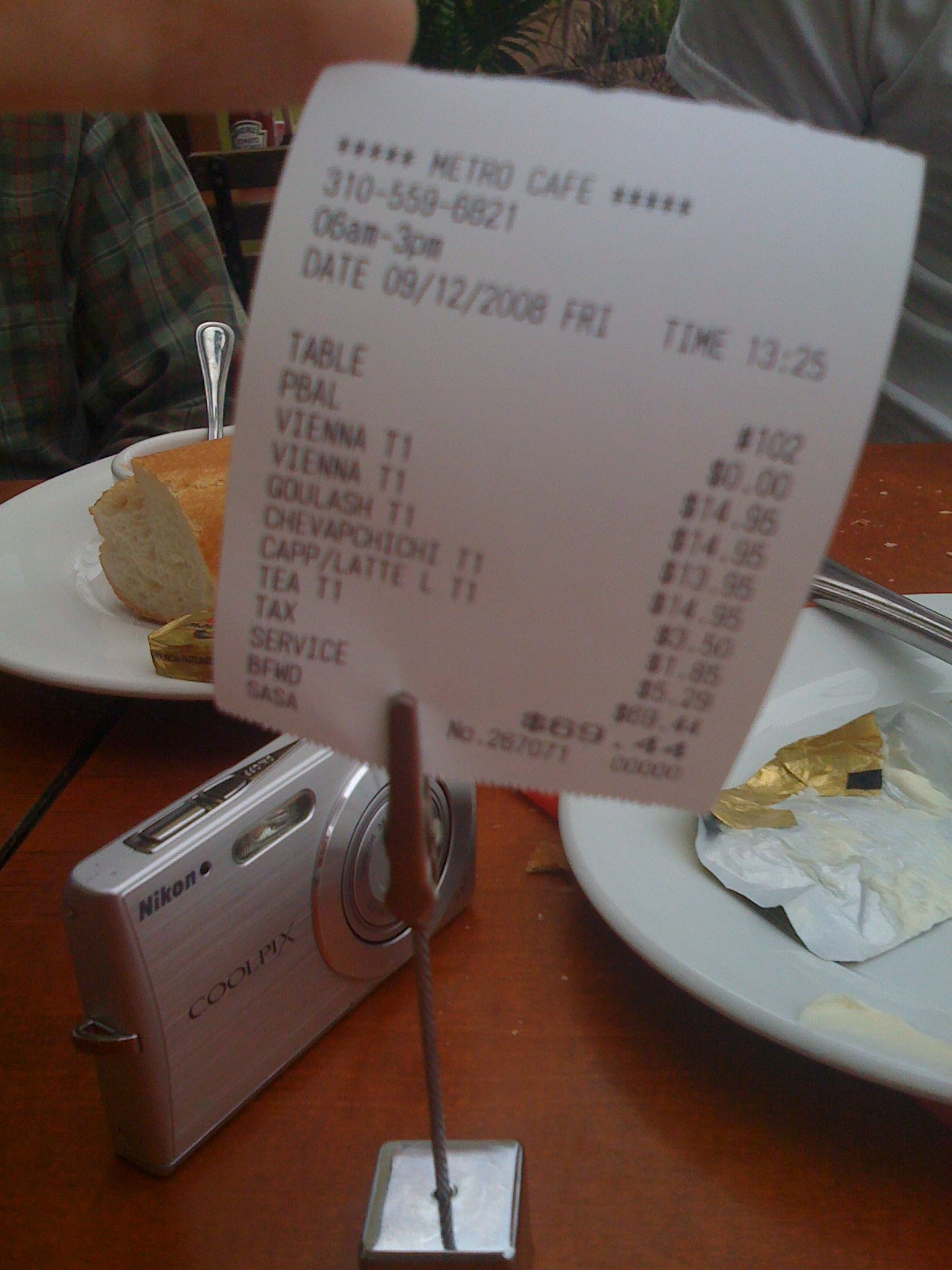This is a detailed close-up photograph of a receipt attached to a small metallic holder on a reddish-brown wooden table. The receipt, marked with “Metro Café” bordered by asterisks, contains a phone number, date from 2008, business hours, table number, ordered items—many in Spanish or Italian—and the total charge of 6,944, including tax. To the left, a silver Nikon Coolpix camera is centrally positioned on the lower part of the image. To the right of the camera is a white ceramic plate holding an empty, golden butter foil with some butter smears and a silver knife handle across the plate. Partially obscured by the receipt, another white plate contains a loaf of bread with an unopened butter packet in golden foil. In the background, a small bowl with a spoon sticking out is visible, along with the flannel-shirted upper body of one person on the left and the gray-shirted torso of another person on the right. The focus of the photograph is primarily on the table items, while the receipt is slightly out of focus.